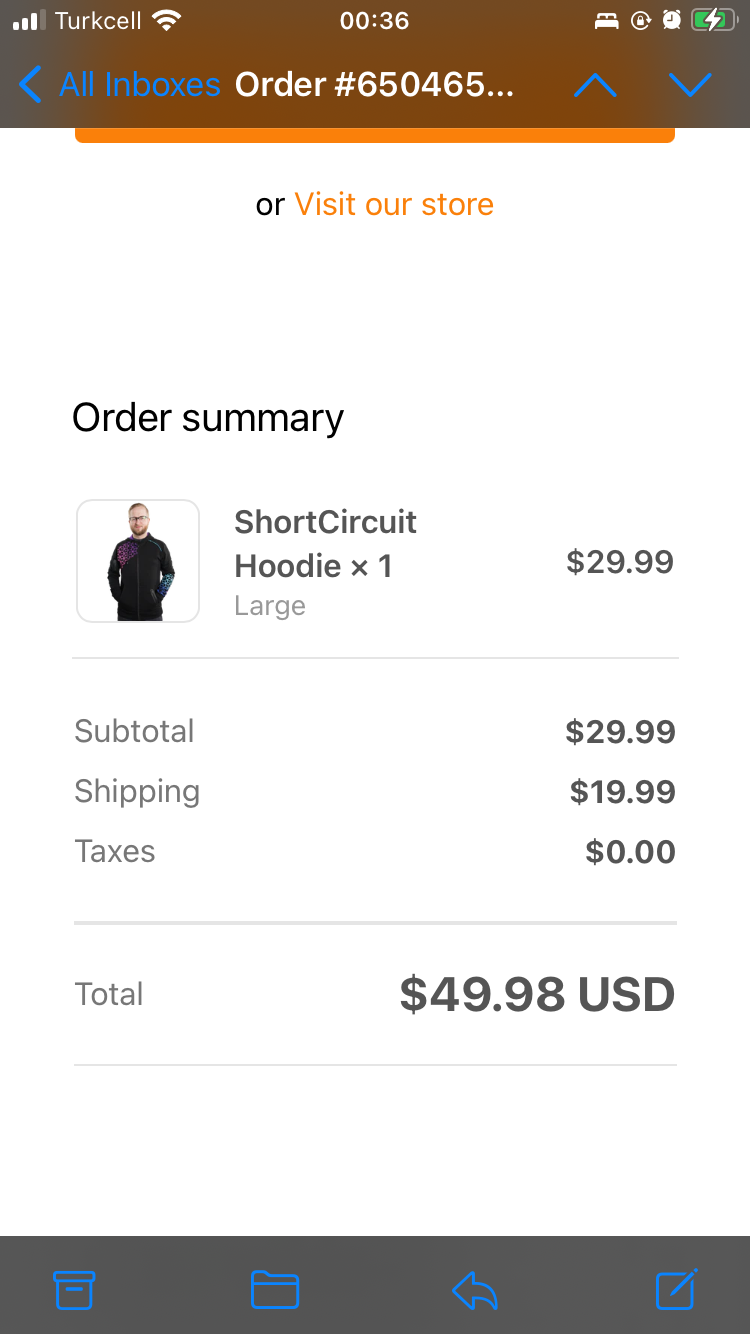The screenshot depicts a military-time-stamped smartphone screen, displaying the order summary from a clothing website. The time is 12:36 AM, indicated as 0036, and the phone is connected to the Turkcell carrier with excellent signal strength, missing only one bar for data. The device is currently charging, evident by the white lightning bolt inside the green battery icon. The order number, partially visible as "650465...", suggests that the user is viewing an order summary page. The item listed is a "Short Circuit Hoodie" in size Large, priced at $29.99. The subtotal for the order is $29.99, with an additional $19.99 for shipping, bringing the grand total to $49.98 USD. No taxes were applied to this order.